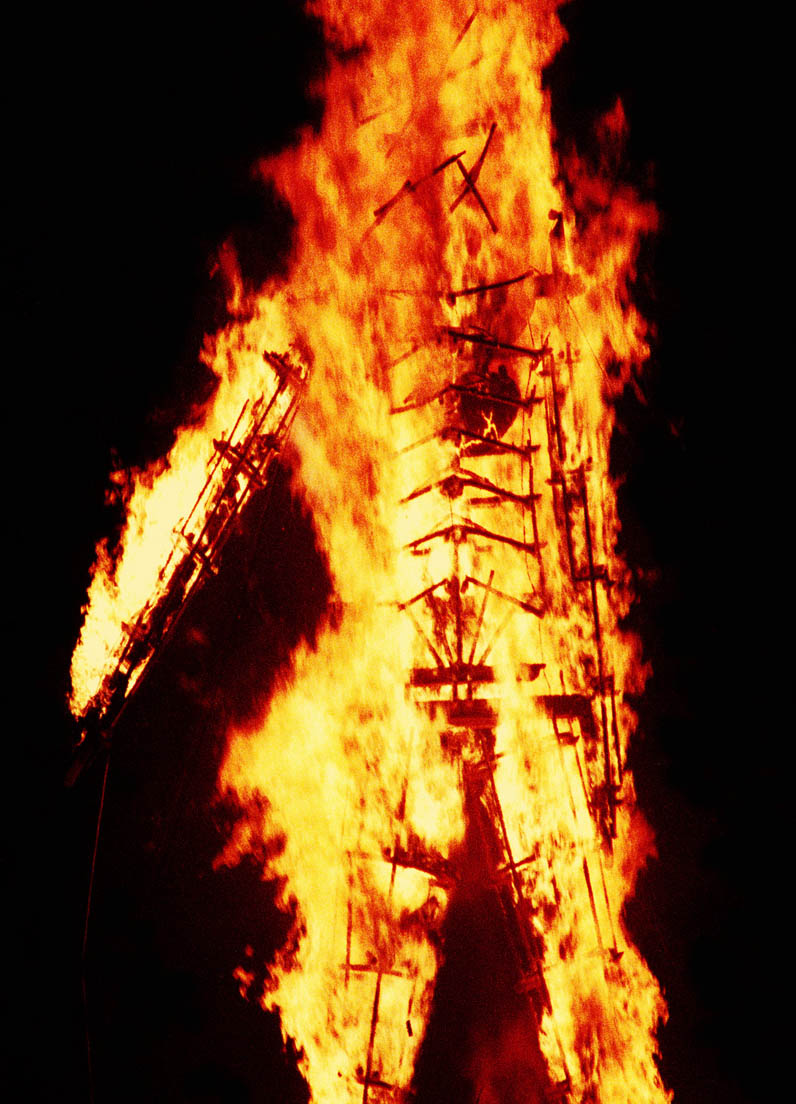The image depicts a towering, human-shaped structure that is completely engulfed in flames against a pitch-black night sky. The fiery figure, resembling a person with a head, torso, arms, and legs, appears to be constructed from wood. The vivid inferno reveals intricate details, including a skeletal form with visible ribs and a defined pelvic area. The fire produces a stunning array of colors—from intense white and yellow flames highlighting the torso to deep red and orange hues crowning the top. One arm is raised at an angle, while the other hangs down by the side, adding to the lifelike silhouette. As the blaze rages, the entire structure and its fiery details—the limbs, connecting joints, and skeletal features—are dramatically illuminated, standing out starkly against the inky darkness.